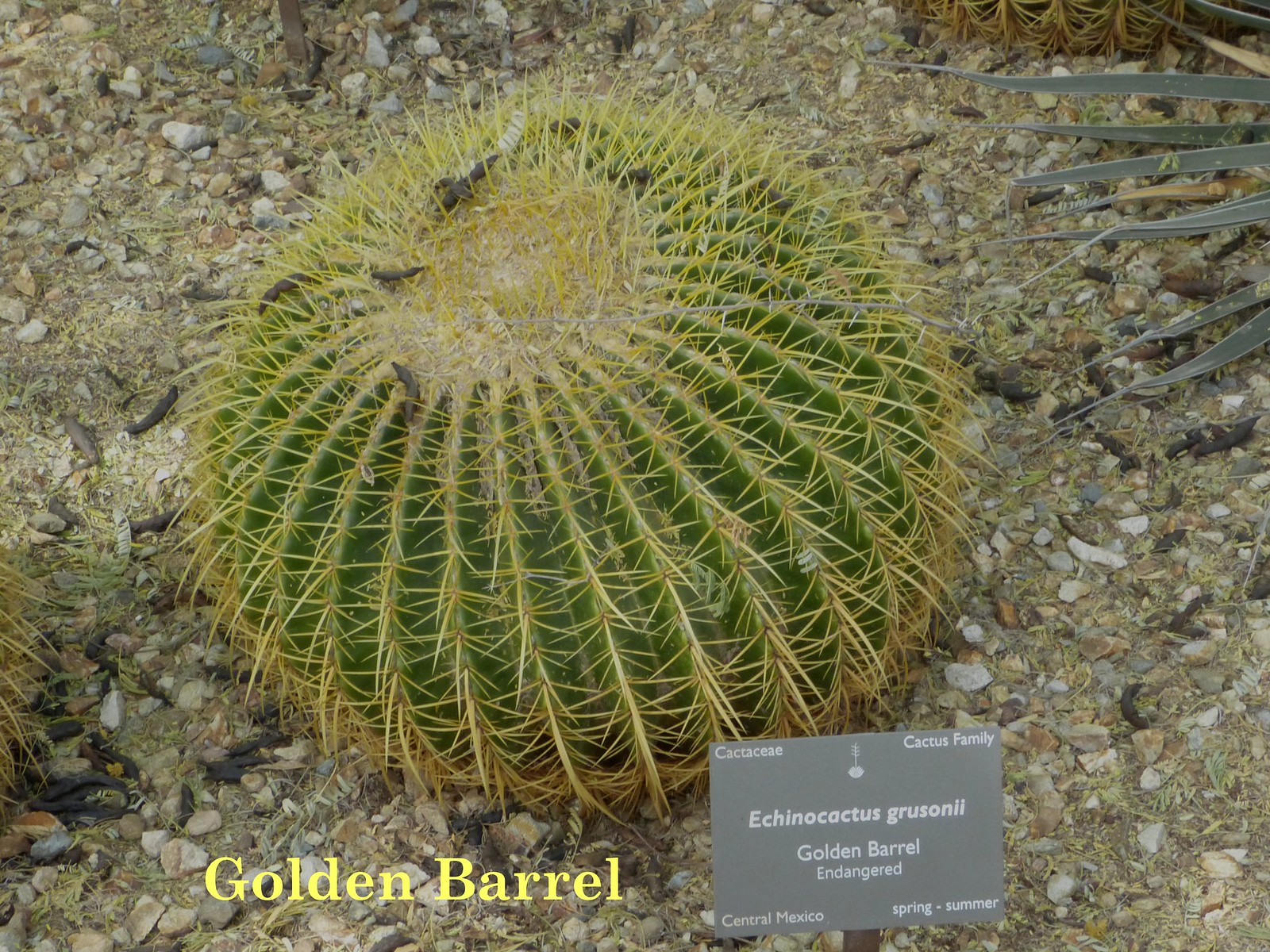This outdoor photograph captures a striking close-up of a green globe-shaped cactus known as the Golden Barrel (Echinocactus grusonii). The cactus is studded with numerous yellow-green spines and rests on a gravelly surface comprised of black and gray pebbles. A business card-sized gray sign in front of the cactus provides detailed information, reading "Cactaceae - Cactus Family, Echinocactus grusonii, Golden Barrel, endangered, central Mexico, spring, summer." In the upper right corner of the image, a hint of another plant's petals can be seen. Additionally, the text "Golden Barrel" is imprinted in yellow on the photo.